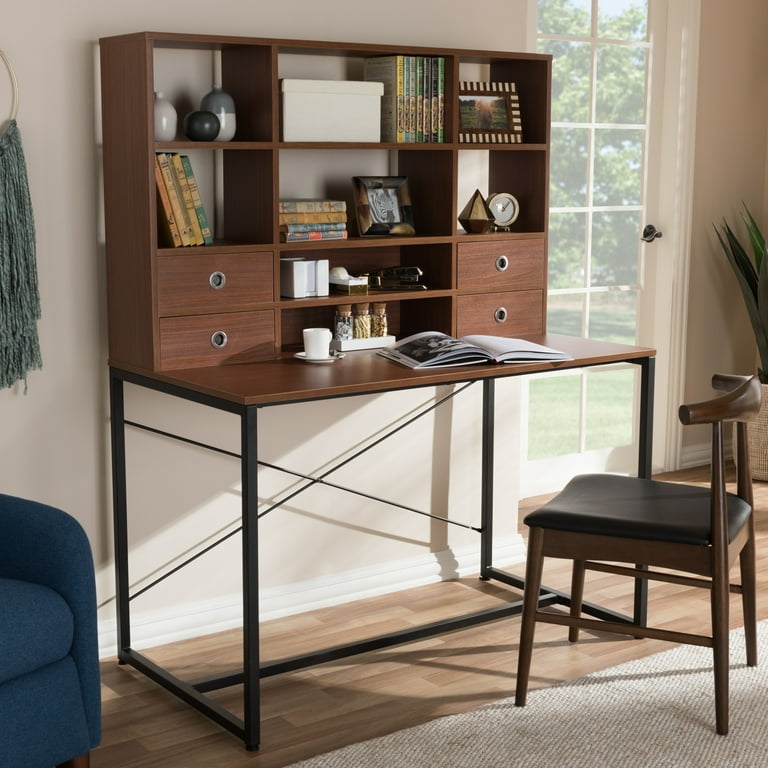The image depicts a well-organized home office setup centered around a mid-century modern wooden desk with a brown tabletop and contrasting black metal legs, which are interconnected with a black rod and crisscross design at the back for stability. The desk features an intricate shelving unit that includes six open compartments arranged in two rows of three above, allowing visibility through to the wall behind, alongside two closed drawers at the bottom and an additional shelf space in the middle, which also has a backing. This workspace is meticulously arranged with decorative elements such as vases, books, a clock, framed pictures, and small vials containing natural materials. On the desktop, a white teacup and saucer and an open book are neatly placed. In front of the desk, there is a wooden chair with a walnut finish and a black seat cushion, complementing the desk's modern aesthetic.

To the left side, the image partially shows a medium dark blue sofa indicating a relaxing area, possibly for breaks. On the right side, there's a slightly open door with white paneling and a large glass window, revealing a lush green outdoor view, adding a touch of nature to the room. A houseplant is also seen near the door, enhancing the room's serene ambiance. Above the blue sofa, there appears to be some green macrame hanging, adding an artistic flair to the space. The overall composition of the room suggests a perfect blend of functionality and aesthetics, conducive to both work and relaxation.